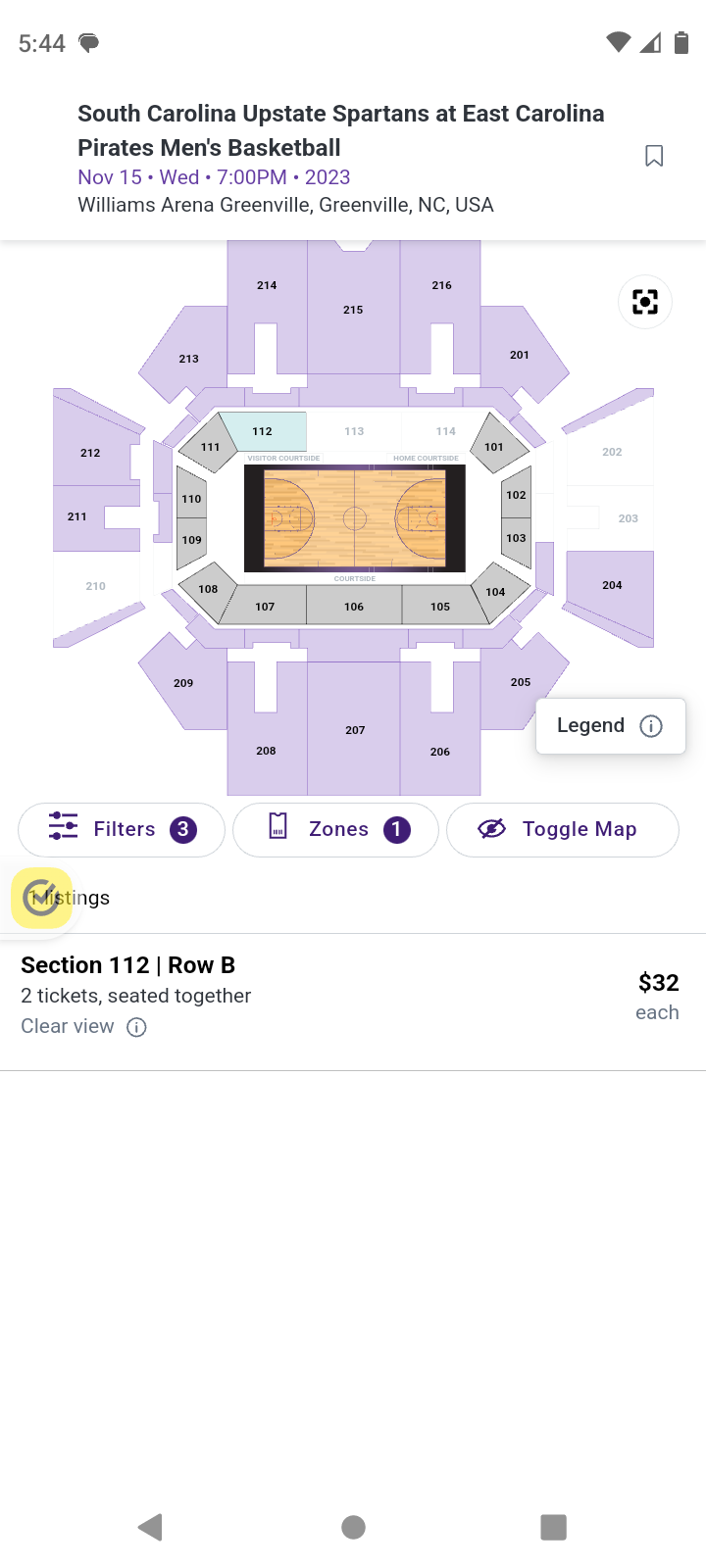Digital screenshot of a basketball event: The image features a detailed layout for purchasing tickets to a men's basketball game between the South Carolina Upstate Spartans and the East Carolina Pirates. The game is scheduled for Wednesday, November 15, 2023, at 7 p.m. and will be held at Williams Arena in Greenville, North Carolina, USA. The seating chart of the stadium shows sections numbered 214, 215, 216, 201, 209, 208, 207, and 206. Highlighting available seating, section 112, row B, offers two tickets seated together with a clear view of the court. The price for each of these tickets is listed at $32.